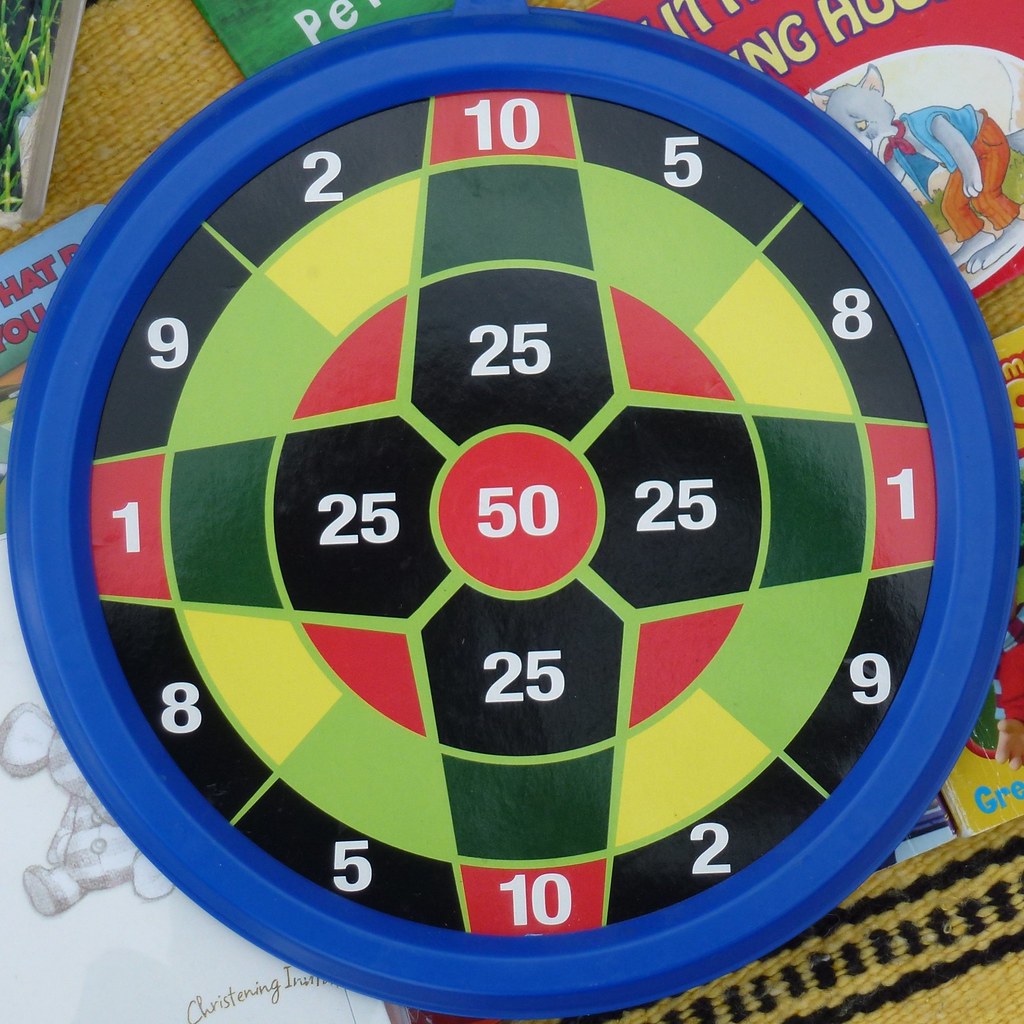The photo features a circular, dart-style target board designed for a different game. The board is segmented into various zones, each marked with different point values. At the center of the board, the bullseye is prominently labeled as worth 50 points. Surrounding the bullseye, there is a concentric ring where hitting any part earns 25 points. The outer regions of the board are divided into multiple sections with point values ranging from 1 to 10. Points are distributed as follows: 10 points zones are located at both the top and bottom, while the sides feature 9 and 8 point zones. Additionally, there are sections marked with 5, 2, and 1 points on the left and right sides respectively.

Among the clearly marked numerical zones, some areas near the center are color-coded but not specifically labeled with point values. These zones are red, yellow, and green, adding a splash of vibrant colors to the middle area of the target. The game's scoring appears to be visually detailed and complex, offering a variety of point-earning opportunities depending on where the player’s marker lands.